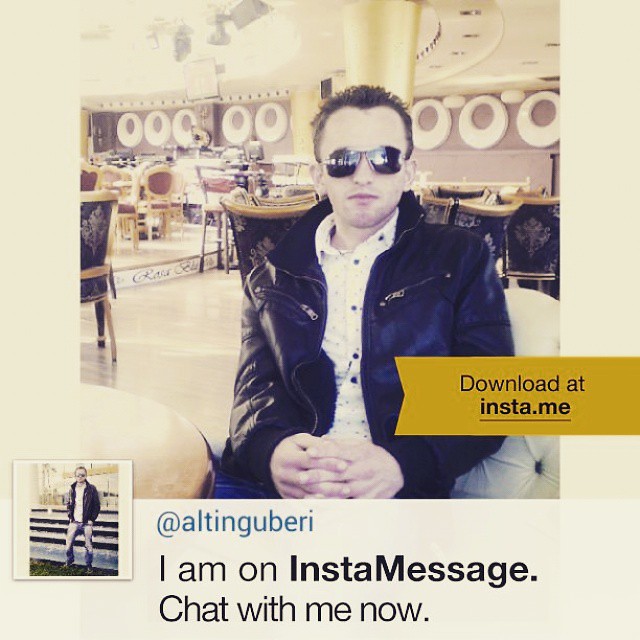The photograph depicts a white gentleman with short spiky hair and dark sunglasses obscuring his eyes. He has a one-day shadow beard and is dressed in a black leather jacket. Seated in a white embroidered chair with a floral design and a black back, his hands are folded in his lap. The setting behind him appears to be a restaurant or showroom, featuring multiple chairs and tables, and possibly a small stage to the left. 

An orange-gold ribbon to his left reads “Download at insta.me,” and additional text at the bottom of the image states “At @altingubri. I am on instant message. Chat with me now.” This message is displayed above a light tan brown background. Adjacent to this message is a smaller thumbnail image of the same man in the same outfit, standing in a field and looking directly at the viewer.